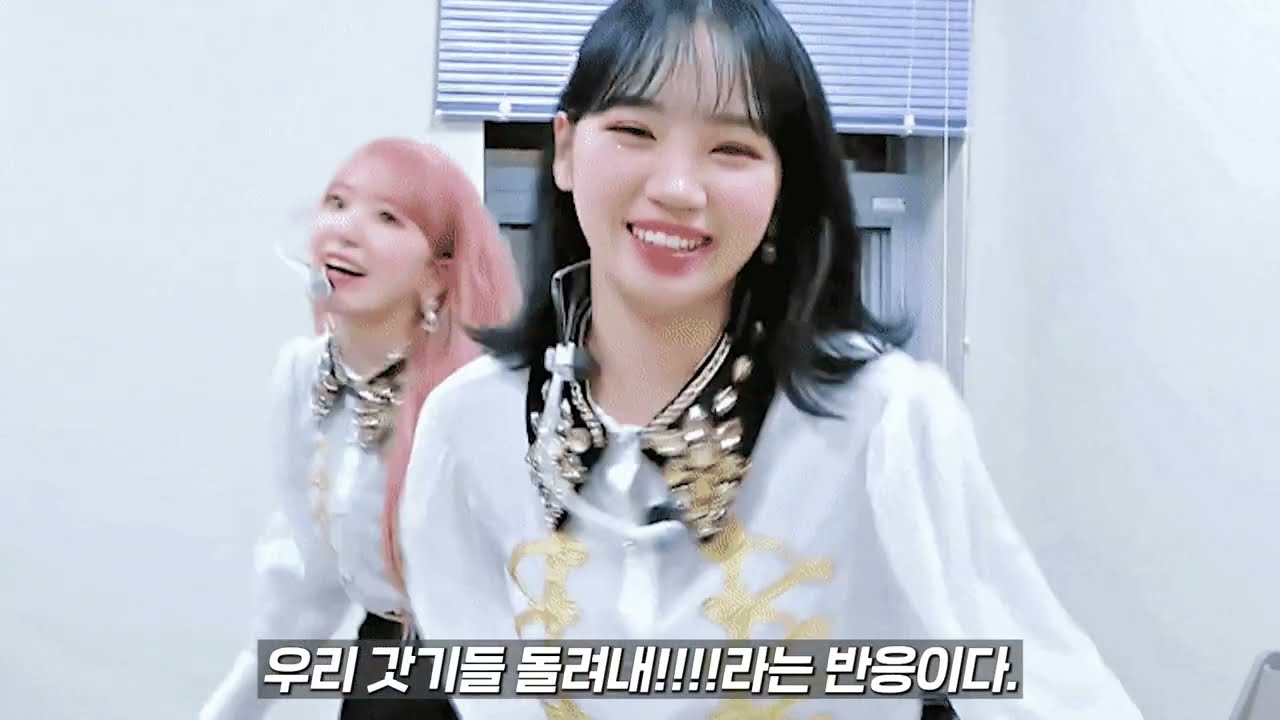In this detailed horizontal rectangular photograph, two Asian women are standing in a room with white walls and a window behind them, the blinds pulled up revealing the cords. Both women are smiling. The woman in the foreground has straight, shoulder-length black hair with bangs, and she is showing her teeth as she smiles. She is adorned in a long-sleeve white blouse featuring a gold pattern on the front and a black collar embellished with gems. 

In the background, slightly blurry, stands the second woman with long, pink hair and bangs, also wearing an earpiece and a microphone at her chin. She is dressed in an identical white blouse with the ornate black and gold-studded collar. 

At the bottom of the image are unreadable white symbols highlighted against dark gray rectangular backgrounds, potentially in South Korean or Chinese. The composition and attire of both women give a hint that they might be pop stars, contributing to a lively and professional ambiance.